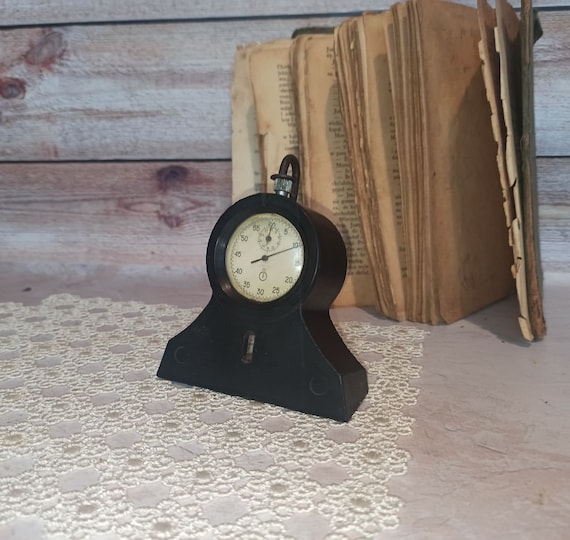In this aged photograph, the focus is on a black, round-faced clock, possibly a barometer, which rests on a white laced doily with widely spaced holes. The clock, appearing small and old-fashioned, is set on a beige cream-colored surface. Behind the clock, there is a visibly ancient and tattered book; its brown, dingy pages are splayed out, some torn and falling apart, indicating significant age and disrepair. A light-colored wooden background with some dark brown knot holes complements the scene, enhancing the vintage and weathered ambiance. The entire composition exudes an antique charm, captured amidst the aged wood grain of the planks that resemble old house paneling.